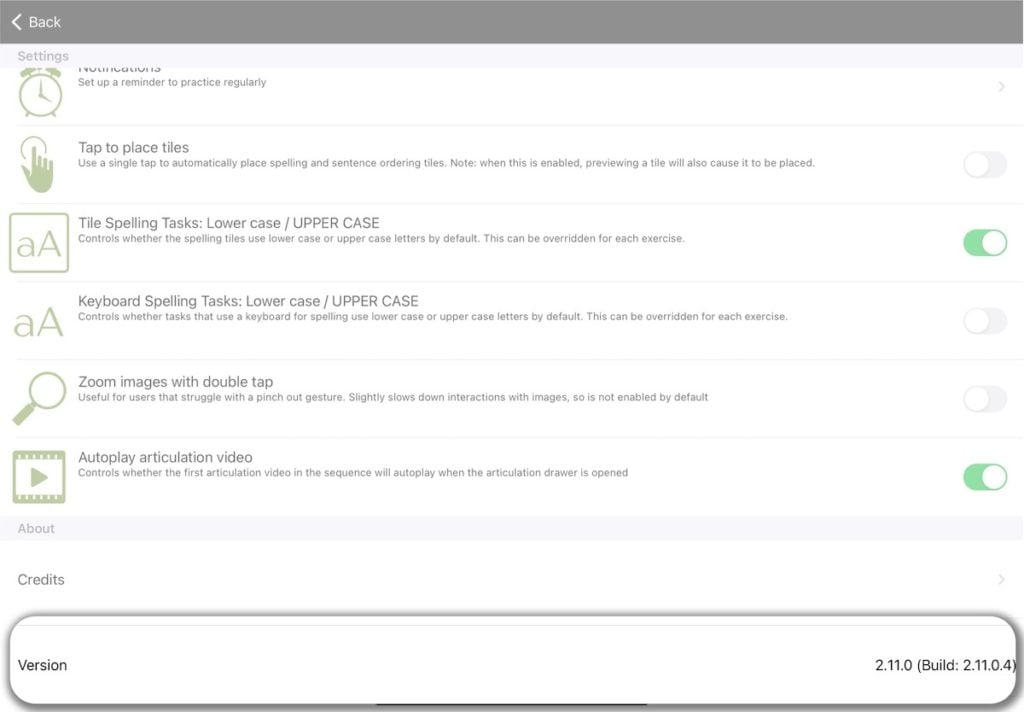This image captures a detailed view of a settings screen interface. At the very top, a thick gray bar contains a back arrow, which sits above a lighter gray bar displaying the title "Settings." Below this, an alarm clock icon is visible, with partially obscured text next to it—indicating that the page has been slightly scrolled. The legible part of the text next to the clock reads, "Set up a reminder to practice regularly."

Further down, several options are listed:

- "Tap to play titles"
- "Tile spelling tasks: lowercase, uppercase"
- "Keyboard spelling tasks: lowercase, uppercase"
- "Zoom images with double tap"
- "Autoplay articulation video"

The version information "Version 2.11.0" and the build number are displayed at the bottom of the screen. Notably, the options for "Tile spelling tasks" and "Autoplay articulation video" have been turned on.